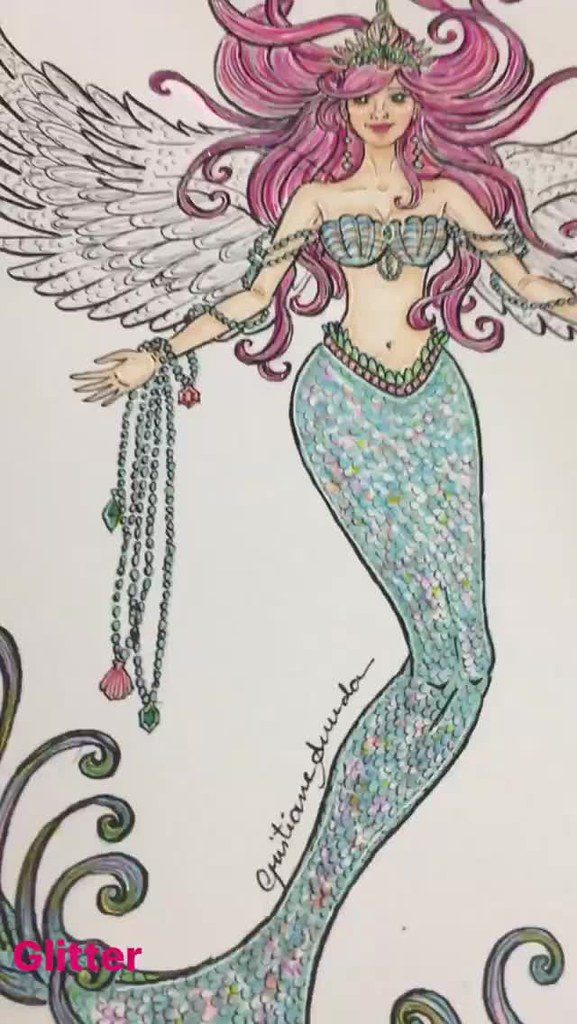This detailed photograph captures a partially colored page from an adult coloring book. The focus of the image is a mermaid, outlined in black ink, that has been creatively brought to life with colored pencils. The mermaid's flowing hair is beautifully shaded in gray, and she wears a delicate crown atop her head. Her skin is rendered in a Caucasian tone, and her torso is modestly adorned with clamshells over her breasts. She also displays ornate chains cascading down her extended left arm, adding a touch of elegance to her appearance. The lower part of her body transitions into a gracefully drawn fish tail, which has an artist's signature placed neatly on it. Interestingly, the mermaid also possesses wings that have yet to be colored in, hinting at the ongoing creative process. The image speaks to the care and detail poured into the coloring and serves as a beautiful snapshot of artistic expression.